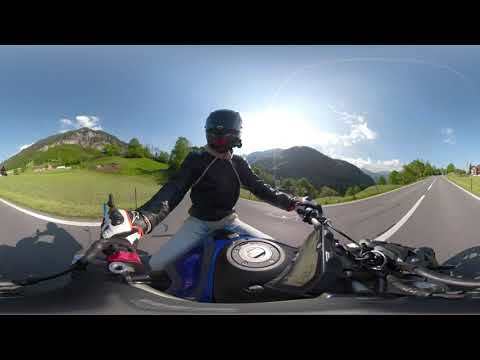In this captivating photograph, a biker is seen riding a black motorcycle on a curving road, captured with a fisheye lens that gives the image a distinctive curved appearance. The biker, centrally positioned in the frame, dons a black helmet, a black jacket, and light blue jeans, with black and white gloves gripping the handlebars of the motorcycle. The road, a greyish hue marked with white lines, stretches prominently across the image, merging dynamically with the surroundings due to the lens effect. On either side of the road, lush green grass blankets the ground, leading the eye towards distant brown mountains. To the left, the landscape slopes gently upwards, while more prominent hills or small mountains rise to the center-right. Above, a clear blue sky is dotted with white clouds, and a bright, white sun is partially obscured by one of the mountains, casting a sizeable shadow. The overall scene combines the thrill of motorcycling with the serene beauty of the natural landscape.